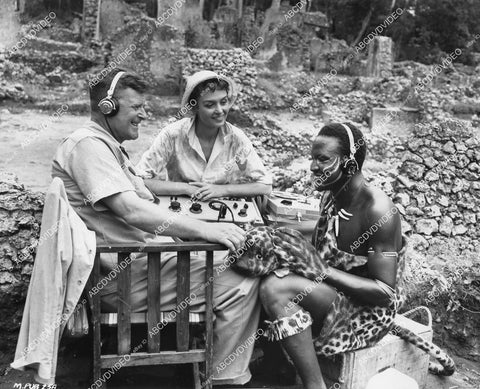In this black and white photo, a seemingly anthropological scene unfolds featuring a European Caucasian couple and an African native man engaged in an intriguing cultural exchange. The African man, dressed in traditional garb that includes a loincloth made of lion's fur and leopard skin accents around his chest and calves, sits on a basket. He sports tribal markings on his face and a headband, which appears to be a pair of headphones connected to a machine held by the couple seated opposite him on wooden slat chairs.

The Caucasian woman, wearing a white hat and a short-sleeved blouse with a collar, smiles warmly at the African man. She sits with her hands on an audio panel, likely demonstrating its use. The Caucasian man, in a short-sleeved shirt and light-colored trousers, also smiles at the African man, sharing the experience through another pair of headphones. His white jacket is draped over the back of his chair.

The backdrop of the image reveals a series of stone structures and pillars, resembling old ruins that create a sense of historical or archaeological significance. The mood is one of connection and curiosity, as both the couple and the African man share a moment of technological introduction against a backdrop of foundational, unfinished stone structures.